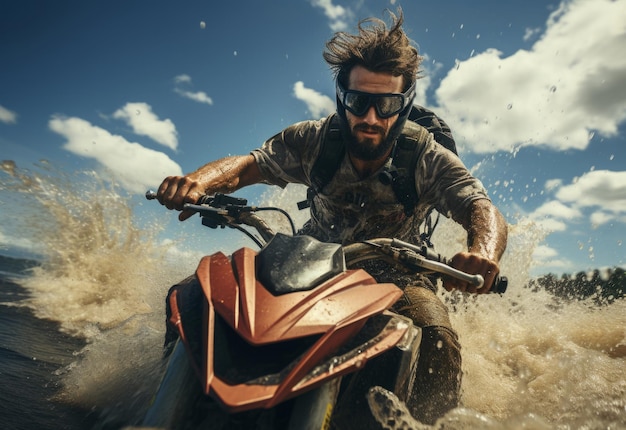The image depicts a highly detailed and photorealistic man with short, wild, wind-blown brown hair riding an orange and black jet ski through muddy, splashing water. He has a pair of mirrored goggles that obscure his eyes and add an air of determination to his expression. His attire comprises a dirty, possibly camouflage shirt, brown pants, and a black backpack on his back. The man’s strong, tan forearms are visible, gripping the handlebars of the speeding jet ski. His wet clothing indicates the intensity of his ride. The background showcases a vibrant blue sky, dotted with fluffy white clouds, and distant trees along the shoreline. The overall dynamic of the scene is enhanced by the waves crashing around him, emphasizing the speed and motion of his thrilling adventure.